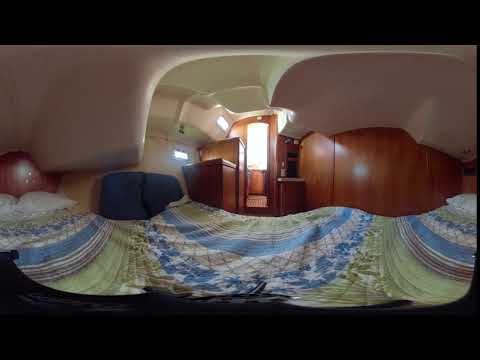The image shows the compact and cozy interior of what appears to be an RV bedroom. The overall space is quite small and rounded, indicative of being inside an RV or possibly a cruise ship cabin. The bed is centrally located, adorned with a multi-colored blanket comprised of green, blue, purple, and white patterns, accompanied by a blue pillow. The wooden walls and cabinetry give the space a warm ambiance, and you can spot a couple of small windows allowing natural light to filter in. 

On the left side of the image, part of the bed and a peculiar, spooky figure with white orb-like eyes can be seen, adding an eerie touch to the otherwise serene setting. The walls are primarily brown, and a door is visible, possibly leading to a compact bathroom with similar wooden paneling. The image, taken from the perspective of someone lying on the bed, captures a midday scene with bright sunlight streaming in. The lack of any visible text adds to the simplicity and functional coziness of the room, highlighting its laid-back atmosphere perfect for travel.